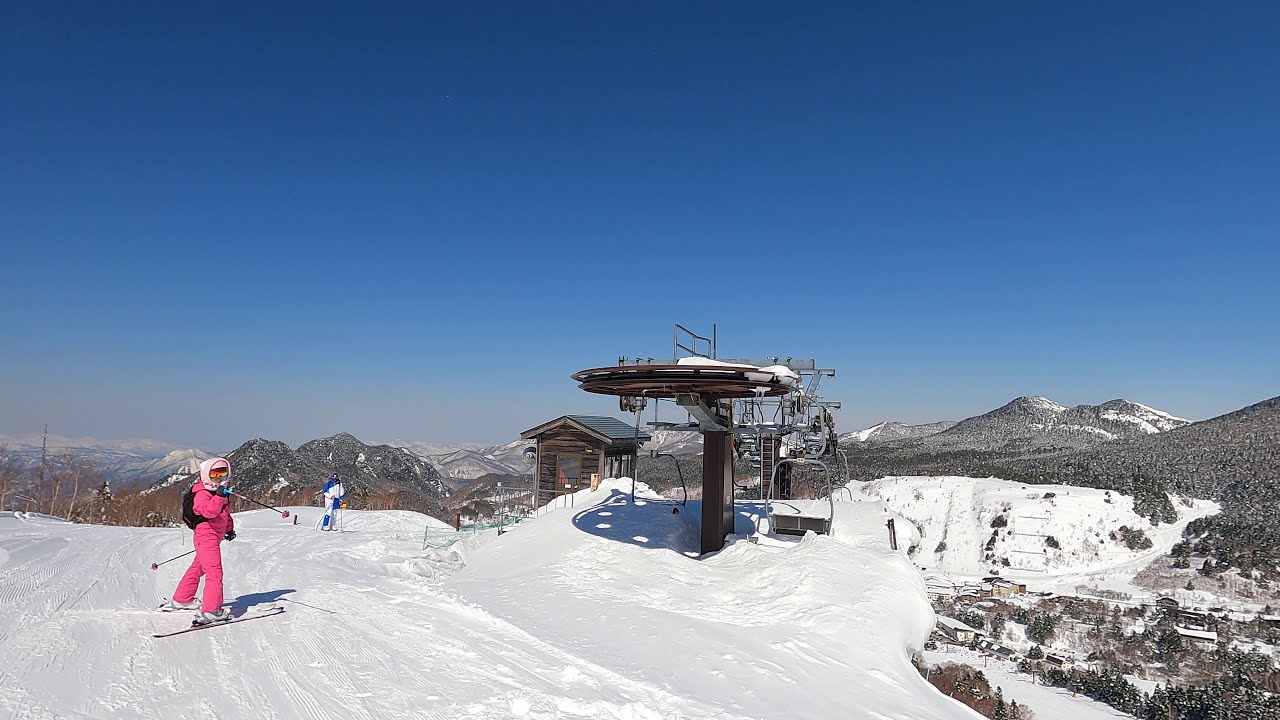In this rectangular outdoor photograph taken at a ski resort high in the mountains, a crisp, clear blue sky dominates the upper two-thirds of the image, stretching down to a horizon lined with scattered mountain peaks. Below, the snow-covered landscape, appearing freshly packed, fills the bottom portion of the frame. In the foreground, ski tracks crisscross the snow, leading to a ski lift station on the right, where empty chairs linger. On the left, a skier dressed in a bright pink snowsuit with a white headpiece and a black backpack stands, looking back at the camera with a smile. Nearby, another skier in a blue and white snowsuit can be seen, positioned further in the distance. Both appear to have recently exited the ski lift, preparing to descend the slope. A small wooden building near the top of the ski lift and a few scattered homes or structures are visible against the picturesque backdrop of mountains and dense clusters of trees, completing this serene winter scene.